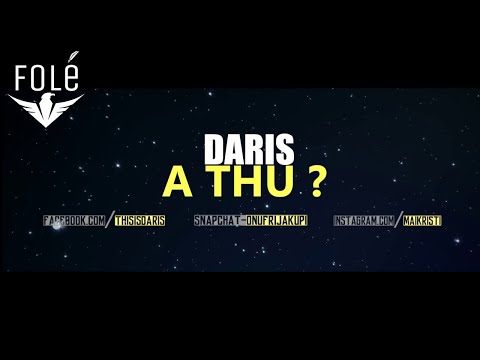The image features a black starry background peppered with small white glowing dots resembling stars. At the top left corner, there is a white emblem of a bird with outstretched wings, alongside the text "FOLE" with an accent over the 'E'. Centered prominently in the middle, "DARIS" is written in large white uppercase letters. Below this, "A THU?" is displayed in yellow uppercase letters. Towards the bottom, the image lists several social media options: "Facebook.com/thisisOris", "Snapchat - ONUFRIJAKUP", and "Instagram.com/MAIKRIST". The entire image appears to be a poster for something potentially related to a popular song on YouTube, given its stylistic design and social media references.